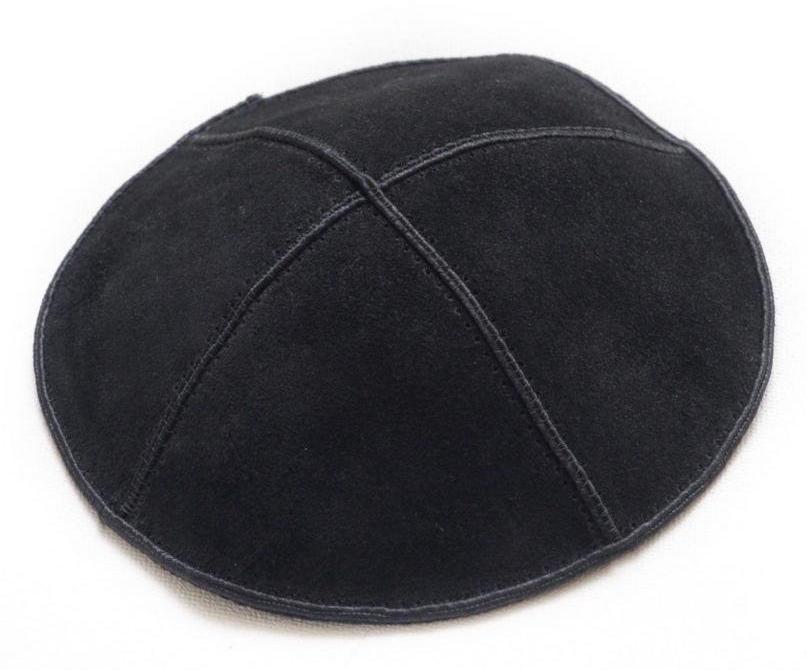The image displays a black yarmulke (or kippah) placed against a white background with a faint shadow on the front left. The yarmulke is crafted from a fabric material that appears to be either felt, suede, or a rough leather-like material. A noteworthy feature is the lighter-colored stitching that forms a cross pattern, creating vertical and horizontal lines across the top and resulting in an X shape. Additionally, there's a seam running around the entire outer edge of the yarmulke, also with a lighter, whiter stitching. The stitching and detailed craftsmanship, including visible holes, suggest the piece is handmade and well-made, with the shiny piping adding contrast against the black fabric.